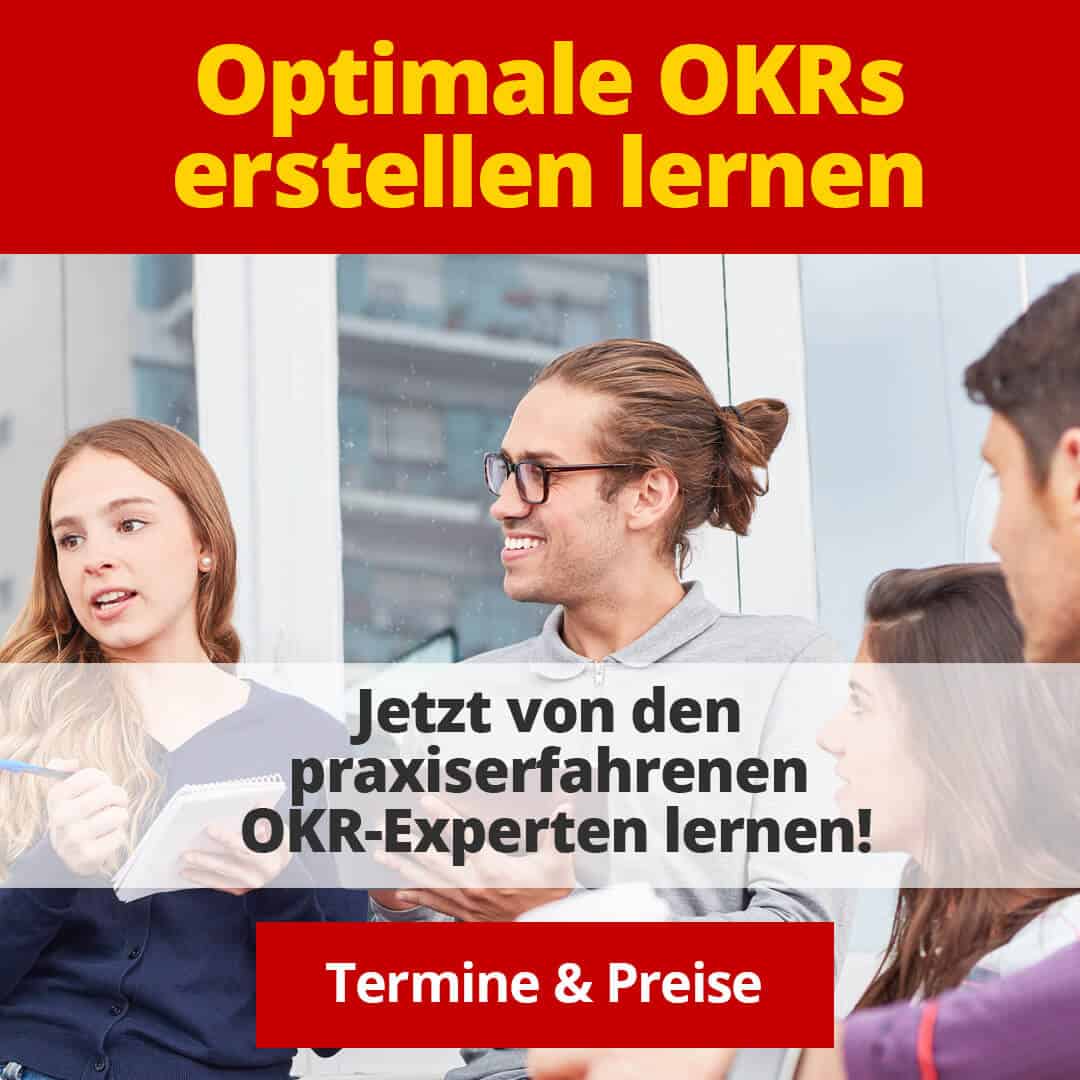The image is an advertisement likely in German, featuring four young adults central to the composition. The subjects include a young woman on the left with brown hair, a blue pen, and a notebook, looking and possibly speaking to the group on the right. In the middle, there's a young man with glasses and a man bun, smiling with his teeth showing, also looking towards the left. To the right, a young woman with shoulder-length brown hair looks attentively at the two central figures, her mouth open as if talking. Partially visible on the far right is another young man with short brown hair. 

The ad is text-heavy, with multiple areas of text in bold colors and strong contrasts. At the top, there's a red box with the yellow letters: "OPTIMAL OKRs ERSTELLEN LERNEN." In the middle, the text reads: "JETZT VON DEN PRAXISERFAHRENEN OKR-EXPERTEN LERNEN!" in black letters on a white background. At the bottom, there is a small red triangular box with the white words: "TERMINE & PREISE." The image appears to promote educational content related to the implementation and learning of OKRs (Objectives and Key Results).